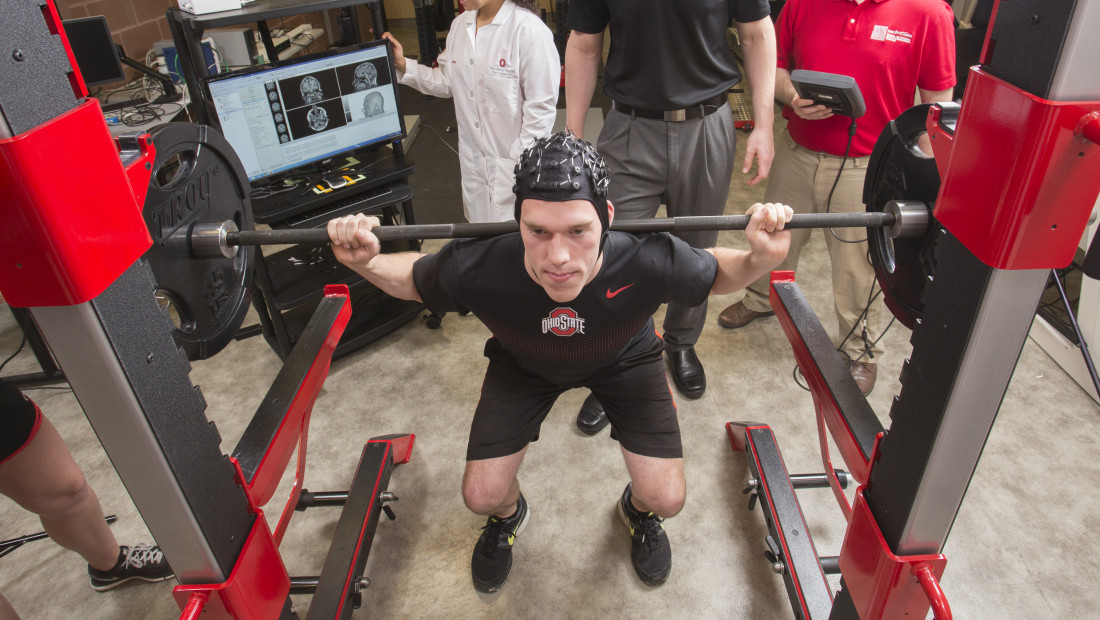In this detailed image, a muscular bodybuilder, outfitted in a black Nike t-shirt, black shorts, and black sneakers, is performing a weighted squat in a laboratory setting. He has a cap on his head adorned with numerous electrodes and sensors. Positioned directly behind him is a spotter dressed in black pants and a black shirt, ensuring his safety. Another individual, dressed in khaki pants and a red shirt, is operating a wired monitor that appears connected to the electrodes on the weightlifter's cap. Nearby, a medical professional in a lab coat stands next to a screen displaying images and data, likely monitoring the bodybuilder’s brain activity during the exercise. Another man, whose muscular legs suggest he is also a bodybuilder, is standing to the left side, possibly ready to assist if necessary. This setting encompasses a sophisticated blend of athleticism and scientific research, focused on understanding the brain's responses to physical exertion.